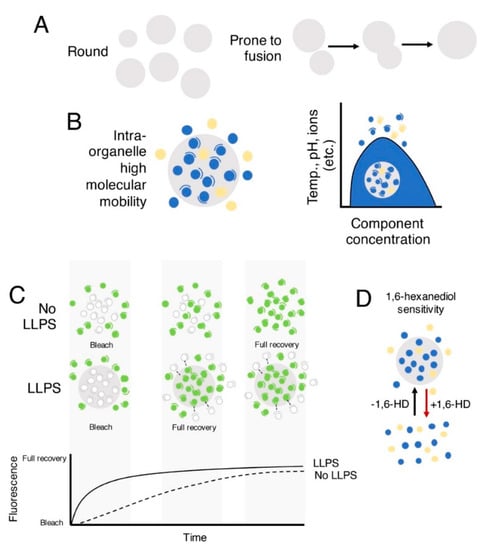This detailed scientific diagram, presented in a cartoon-like format on a solid white background, is segmented into labeled sections A, B, C, and D. On the upper left-hand side, section A features the word "Round" adjacent to six light gray circles, followed by the label "prone to fusion." This is illustrated with two arrows: one pointing from two separate circles to two touching circles, and another leading to a single larger, fused circle. Section B, located below A, is highlighted by the term "intraorganelle high molecular mobility" next to a large light gray circle populated with numerous tiny blue and tan dots. This is accompanied by an L-shaped set of axes labeled "Temp, pH, ions, etc." on the Y-axis and "Component concentration" on the X-axis, showcasing a curved line shaded in blue surrounded by small dots. Moving to the bottom left, section C presents two rows of six images each, the top row labeled "no LLPS" and the bottom "LLPS." Lastly, section D on the lower right indicates "1,6-hexane diol sensitivity," depicted with a large gray circle filled with blue and tan dots. Here, two arrows, one red pointing down and one black pointing up, transition to a background void of the circle but containing the same dot configuration. Another graph in the lower left corner marks “time” on the X-axis and “fluorescence” on the Y-axis, displaying two upward-curving lines.